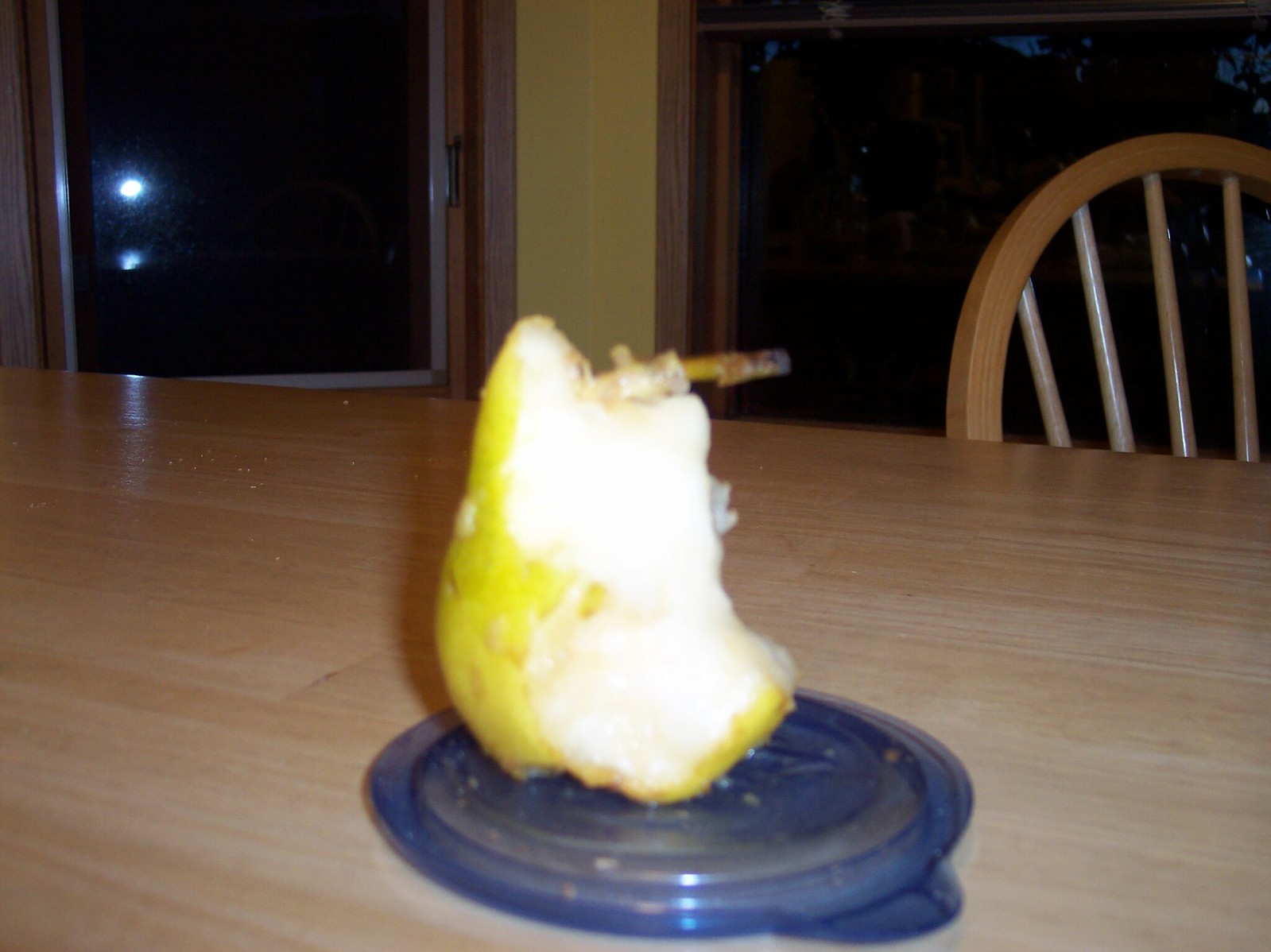The image showcases a partially eaten pear, with approximately three-quarters of the fruit consumed, mostly from the top. The remaining portion, which still has some yellow skin, is placed intact on an inverted blue Rubbermaid container. The pear, centrally positioned, has bite marks around it and a stem that appears to be nearly detached from the core. The Rubbermaid container itself rests on a wooden table, the grain and lines of which are clearly visible. In the background, the upper part of a wooden chair with a half-moon top and protruding spokes can be seen. There's a window behind the chair, designed to slide up and down, while another window with a crank handle is situated to the left of the pear. Sunlight streams through these windows, casting reflections and adding a warm glow to the scene.